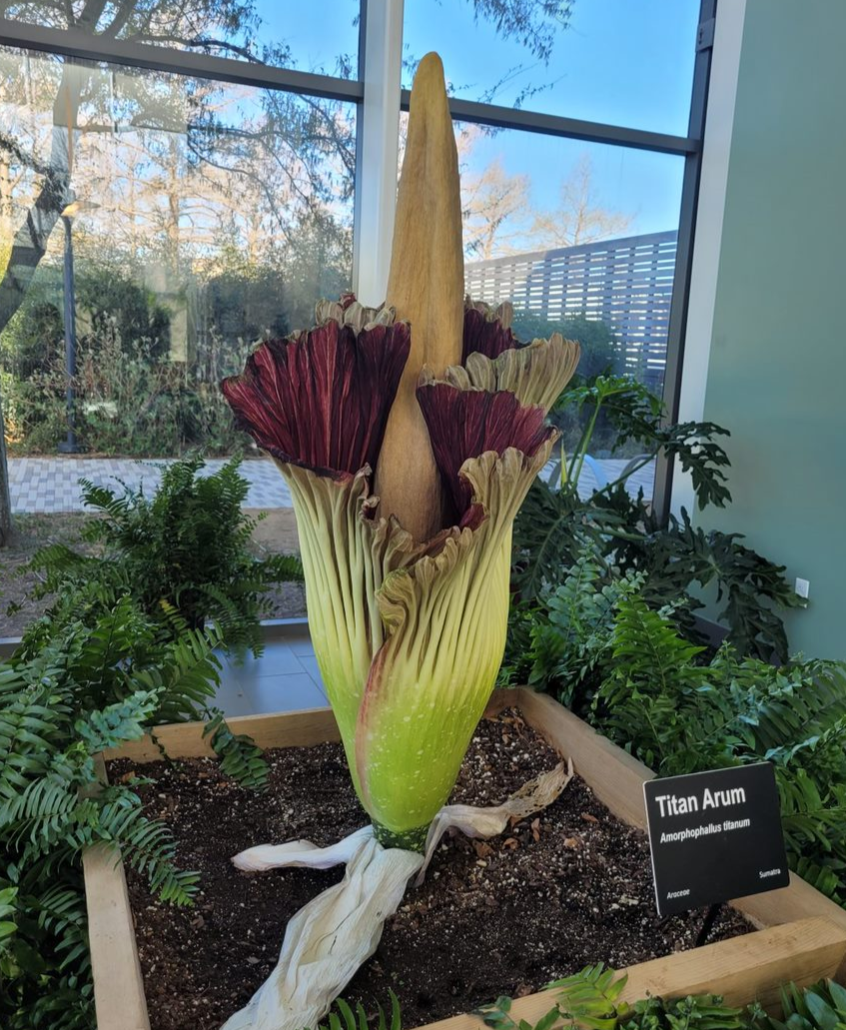The photograph captures a detailed scene of a unique indoor plant exhibit. Central to the image is a large, striking plant situated in a square wooden planter filled with dark brown soil. The plant features lush green, dark brown, and maroon leaves that fold around an orange, tusk-like structure emerging from the center. Notably, three white petals, possibly wilting, can be observed near the base of the plant. The planter bears a small black sign with white lettering that reads "Titan Arum," along with a detailed description in smaller text underneath.

Surrounding the main plant, additional ferns fill the space, contributing to the lush greenery of the setting. The exhibit is placed near a large window with black framing, which offers a view of an outdoor garden area featuring a walkway, other plants, a tree, a fence, and a low gray retaining wall. The sky, visible through the window, is a clear blue, providing a serene backdrop to the indoor scene. The room itself has gray walls, further enhancing the focus on the vivid plant display.